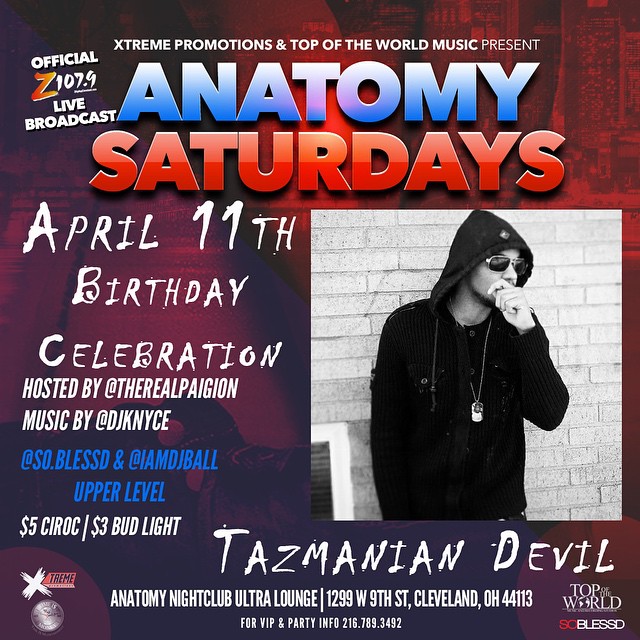This is a square digital advertisement for an event titled "Anatomy Saturdays." The background is shaded completely red, contributing to an indistinct image that appears to be a room or a city. At the top, it reads in white capital letters, "Extreme Promotions and Top of the World Music Present." Below this, the event title "Anatomy Saturdays" is prominently displayed, with "Anatomy" in chunky blue all-caps and "Saturdays" in bold red all-caps.

In the upper left corner, the poster announces in slanted white all-caps, "Official Z107.9 Live Broadcast." Below the main title, to the right, there is a black-and-white photograph of a man in a hoodie, sunglasses, and a dog tag necklace, standing against a light brick wall. His left hand is raised to his mouth, and he is looking to his left.

To the left of the photograph, in white handwriting-like font, it reads "April 11th Birthday Celebration Hosted by The Real Pageon." Further text details the music by DJ Knice and mentions drink specials including $3 Bud Light. At the bottom, the poster features the name "Tasmanian Devil" in a stylized font. The advertisement is visually busy with a mix of white, blue, and red text, mostly in all caps, creating a vibrant, energetic feel.